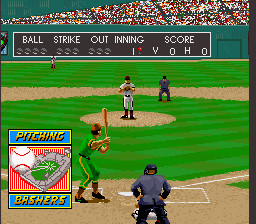This detailed image is a screenshot from a pixelated video game depicting a baseball match. In the foreground, near home plate, a batter dressed in a green and yellow uniform is seen batting right-handed, closely observed by an umpire in all black with his hands on his hips. The backside of another umpire is also visible, standing slightly behind the batter. Positioned on the pitcher's mound in a white uniform is the pitcher, ready to deliver a pitch. Additionally, there is a third umpire positioned out in the field to the right of the pitcher. The field is encompassed by a turquoise colored wall that features a black scoreboard displaying the words “ball, strike, out, inning, score,” with one red light indicating an active strikeout. The scoreboard currently shows a score of zero to zero in the first inning. Above the wall, there is a vibrant crowd filling the bleachers, adding to the lively atmosphere. In the bottom left corner, a box labeled "Pitching Bashers" includes an image of a baseball and a distant stadium, emphasizing the baseball theme of the game. This image captures the essence of the video game from the perspective behind the umpire, offering a comprehensive view of the action and the surrounding elements.